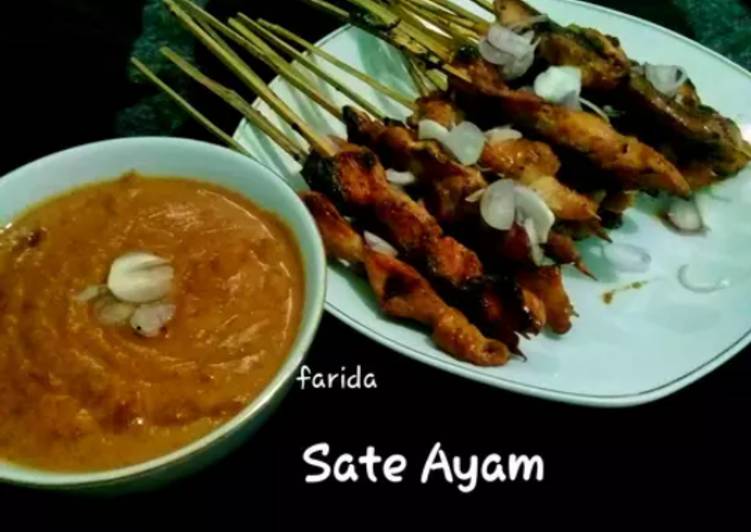The image displays a solid black background with two distinct dishes. On the left, there's a white bowl filled with a thick orange and brown liquid, likely a peanut satay dipping sauce, adorned with a singular white petal or garnish floating in the center. Positioned towards the center-right of the composition, a large, rounded-corner white plate holds several grilled chicken skewers. The skewers, impaled on light brown wooden sticks, are attractively marked with dark grilling lines and are garnished with similar white petals. Between the two dishes, near the bottom of the image, the word "farida" is displayed in lowercase white letters. Directly beneath this, the label "SATE AYAM" is prominently shown in uppercase white letters.